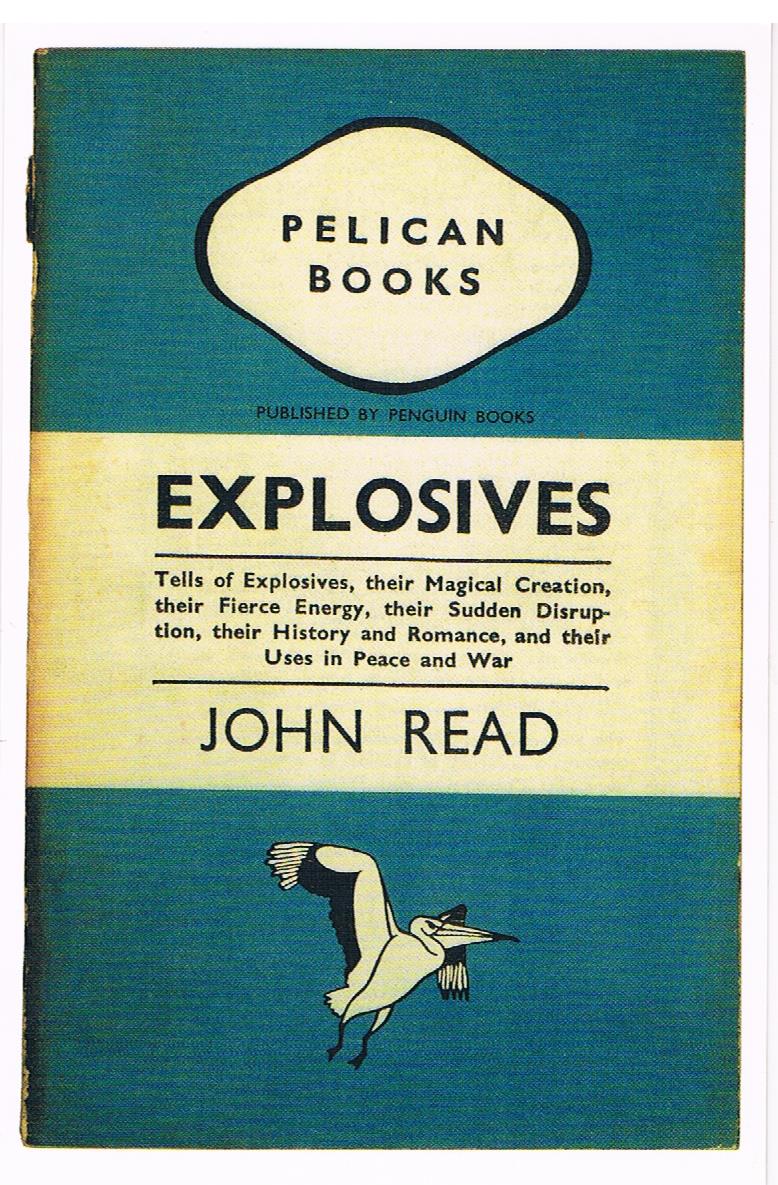This image is a rectangular photograph or scan of a book cover with a dark turquoise or teal background. The cover is divided into three distinct sections. At the very top, there's a white rounded diamond shape with the text "Pelican Books" in black, and just beneath it, in smaller print, "Published by Penguin Books." The middle section features a white band with bold black text that reads, "Explosives." Below this, in smaller font, it says, "Tales of Explosives, Their Magical Creation, Their Fierce Energy, Their Sudden Disruption, Their History and Romance, and Their Uses in Peace and War." The author's name, John Reed, appears at the bottom of this white band. The lower section of the cover returns to the dark turquoise or teal background and includes a black and white illustration of a pelican mid-flight, wings flapping as if about to take off into the sky.